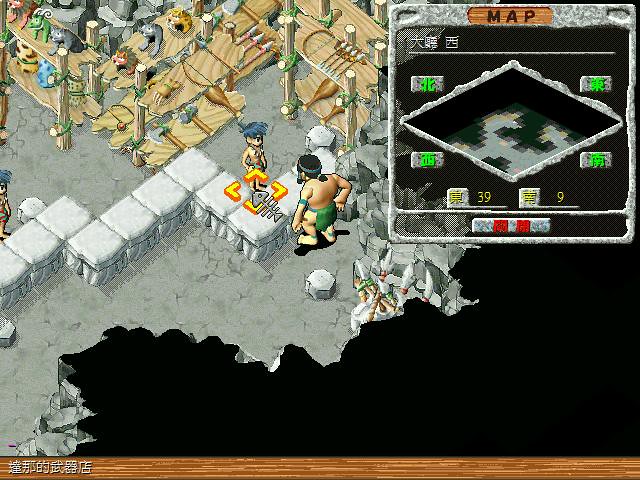This image is a screenshot from a mobile video game, showcasing a richly detailed scene within a tribal setting. At the center, a character that appears to be the main protagonist is depicted from behind. This character, likely male, is minimally clothed, wearing only a simple cloth hanging from the waist and a green arm band. The character's light skin and black hair, paired with another band around the head, further emphasize a tribal aesthetic.

The protagonist is engaging with another character situated behind a row of tiered cement blocks, suggesting this could be an in-game vendor interaction. The NPC being spoken to has distinctive blue hair and is positioned in front of shelves laden with various items, reinforcing the vendor role. The setting is a primitive, cave-like environment with a cement ground that partially appears incomplete, as evidenced by an unrendered black area at the bottom right of the screen.

The game's Heads-Up Display (HUD) features a yellow selection square with orange sides, marked by four brackets at each corner, highlighting a fishbone icon. This element adds to the interaction depth. Below the scene, a brown bar with white lines houses text in an East Asian script, possibly Chinese, Korean, or Japanese, further indicating the game's cultural context. Additionally, in the top right corner, a square with a cement-like border contains a mini-map, displaying various colored areas in greens, grays, reds, and yellows, alongside more East Asian text with a line beneath it.

Overall, the screenshot captures an intricate moment within the game, reflecting a mix of tribal and prehistoric themes combined with modern gaming elements and an East Asian influence.